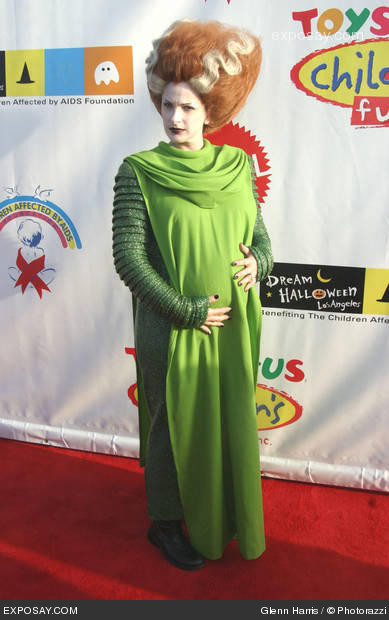In this photo, Marlee Matlin is dressed in an elaborate Bride of Frankenstein costume at a Halloween event. Her outfit features a long green dress with padded, textured sleeves that extend to her wrists, resembling rubbery folds. She sports black nail polish and is cradling her stomach, signaling her pregnancy. Her striking hairdo is a dramatic beehive style, sweeping upwards with bright orange and gray streaks, reminiscent of the iconic Bride of Frankenstein’s look. She poses on a red carpet in front of a backdrop filled with sponsor logos, including Dream Halloween Los Angeles and Toys R Us. At the bottom of the image, white text on a small gray border reads "expose.com" and "Glenn Harris/copyright photo Razzi."